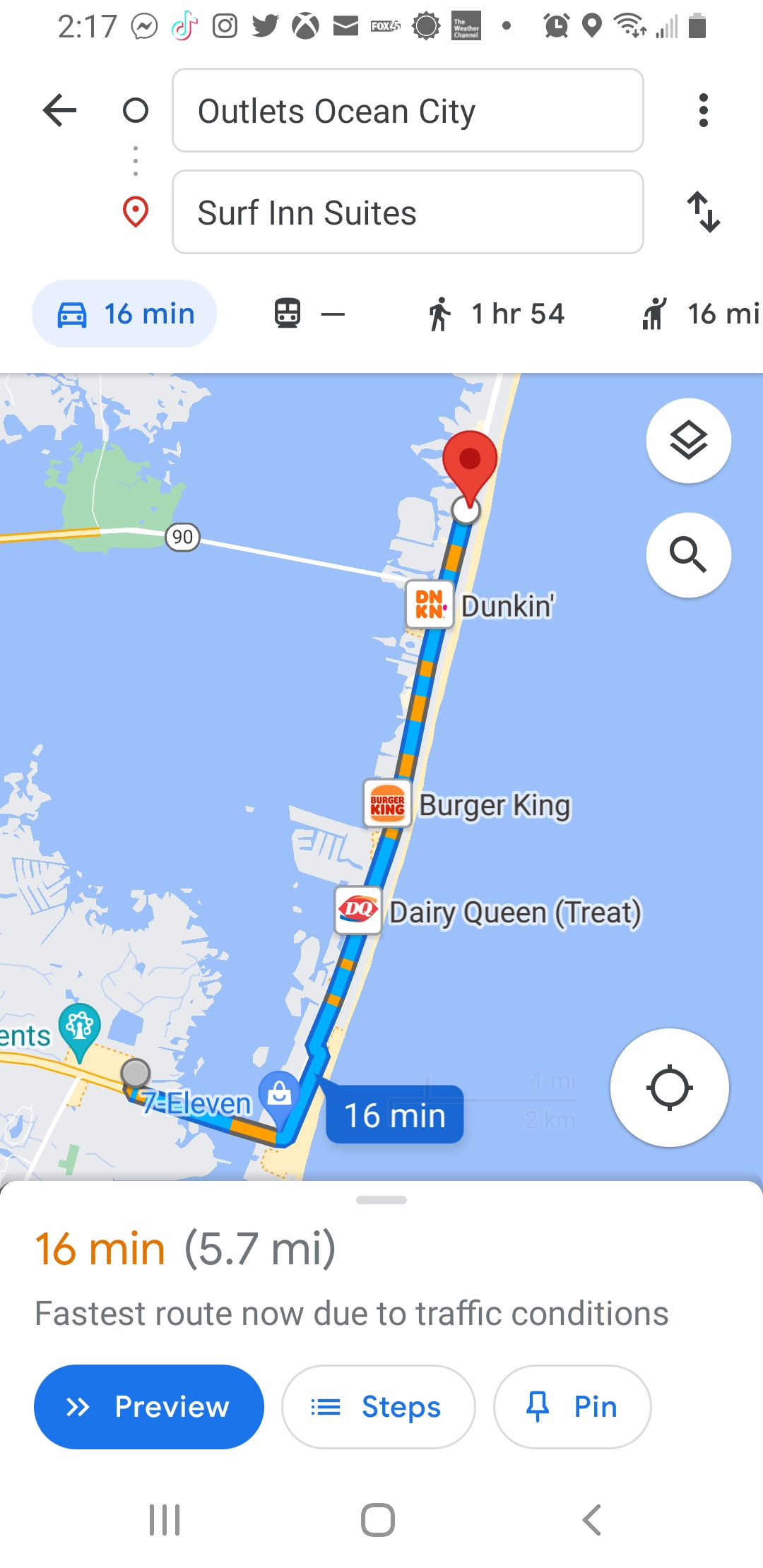A Google Maps screenshot displayed on a smartphone, captured at 2:17 PM, complete with a variety of notifications from Facebook Messenger, TikTok, Instagram, Twitter, PlayStation, email, and weather alerts. The top of the screen shows indicators for an active Bluetooth connection, two bars of cell reception, almost full battery, and an alarm set. The map outlines a route from the outlets in Ocean City to Surf Inn Suites, traversing a narrow strait with water on either side. The journey, spanning 5.7 miles and estimated to take 16 minutes, passes several landmarks including a Dairy Queen, Burger King, Dunkin', and a 7-Eleven near Highway 90. The map also highlights some traffic interruptions along the way. The bottom of the screen provides options to preview steps and access a PIN.